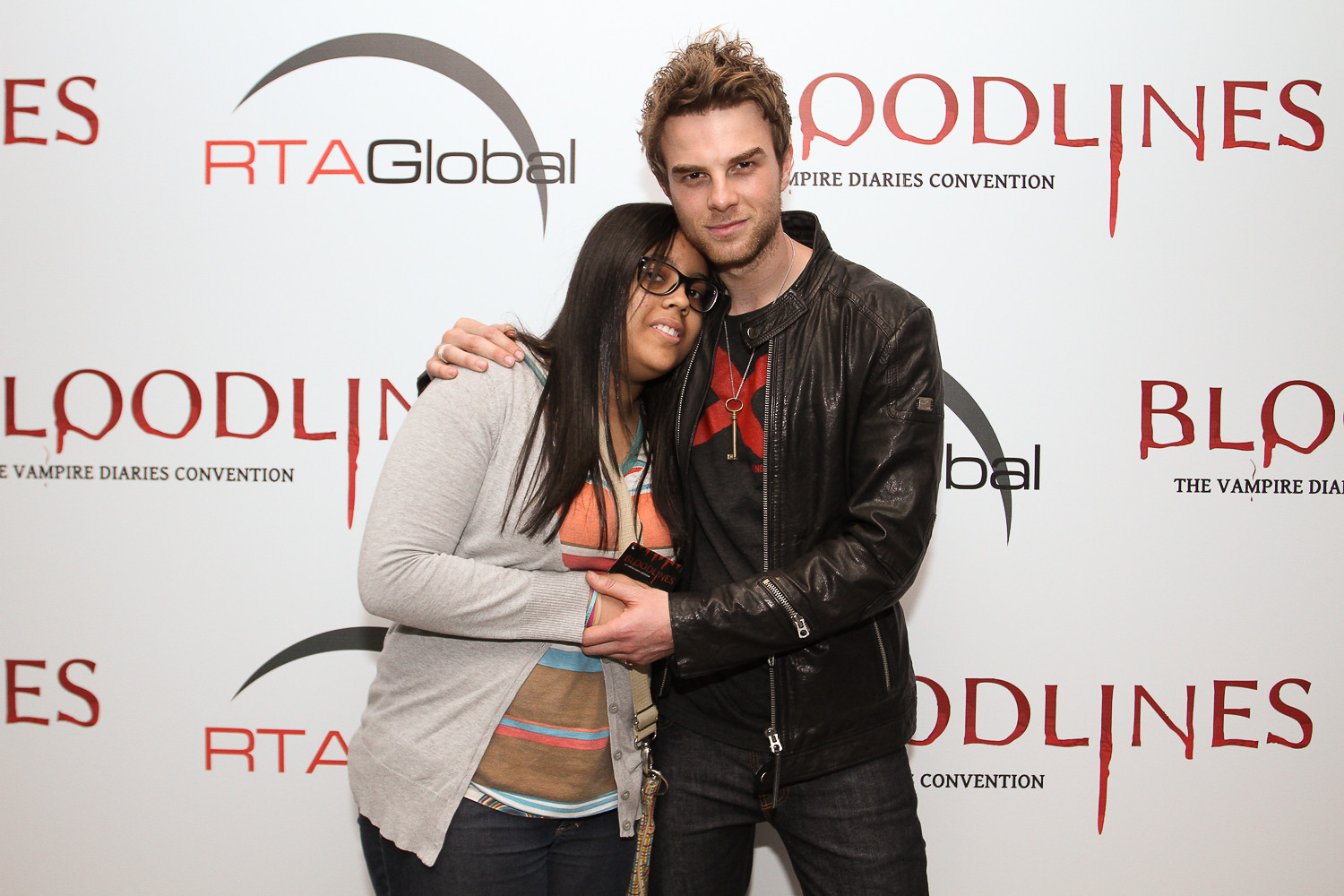In this photograph taken at the "Bloodlines Vampire Diaries Convention," a young man and woman pose together on stage against a backdrop featuring the event's branding and its sponsor, RTA Global, with a distinctive crescent moon logo. The man, positioned on the right, is wearing a black leather jacket, black denim pants, and a gold chain with an old skeleton key. He has blondish hair and a near goatee. The woman, standing on the left, is dressed in a tan cardigan, jeans, and black glasses, with long black hair. The man has his arm around the woman's shoulder, holding her hand, giving the impression of an actor taking a photo with a fan. The event's title, "Bloodlines Vampire Diaries Convention," is prominently displayed in a stylized red font that appears to be bleeding, enhancing the vampire theme of the gathering.